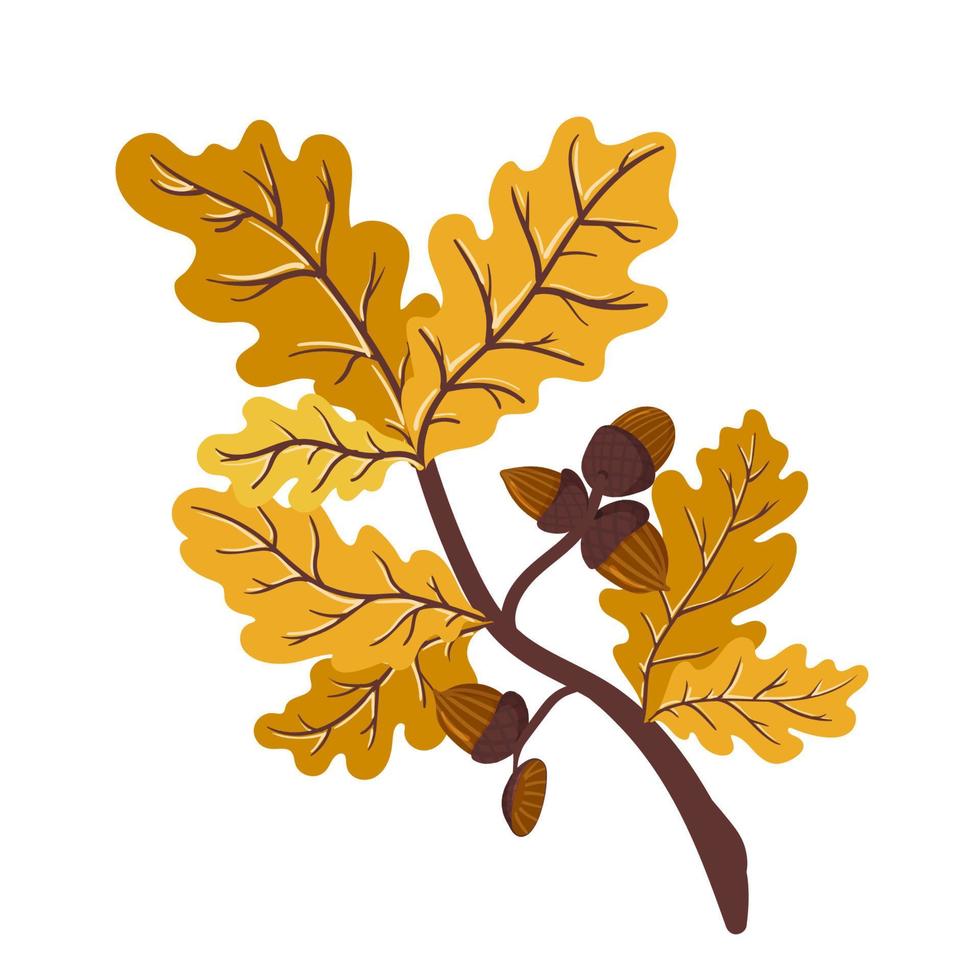This is a clip art style digital drawing of an autumn oak branch. The branch, as thin as a pinky finger, is adorned with seven leaves in a rich autumn palette of orange, yellow, and brown hues, detailed with brown veins. The leaves are arranged in bundles of two to three, specifically with two bundles having one large and one small leaf, and a bundle of three. Additionally, there are four whole acorns and one acorn cap from which the nut has fallen. The acorns themselves have dark brown caps and lighter brown bodies with subtle orange or brownish stripes. In one cluster on the middle right, three acorns remain intact, with two facing upward and one facing downward. Another smaller cluster features a solitary acorn and an empty cap nearby. This image, bearing the clean, simplistic look common to stock icons, provides a versatile autumn-themed element for various graphical applications.